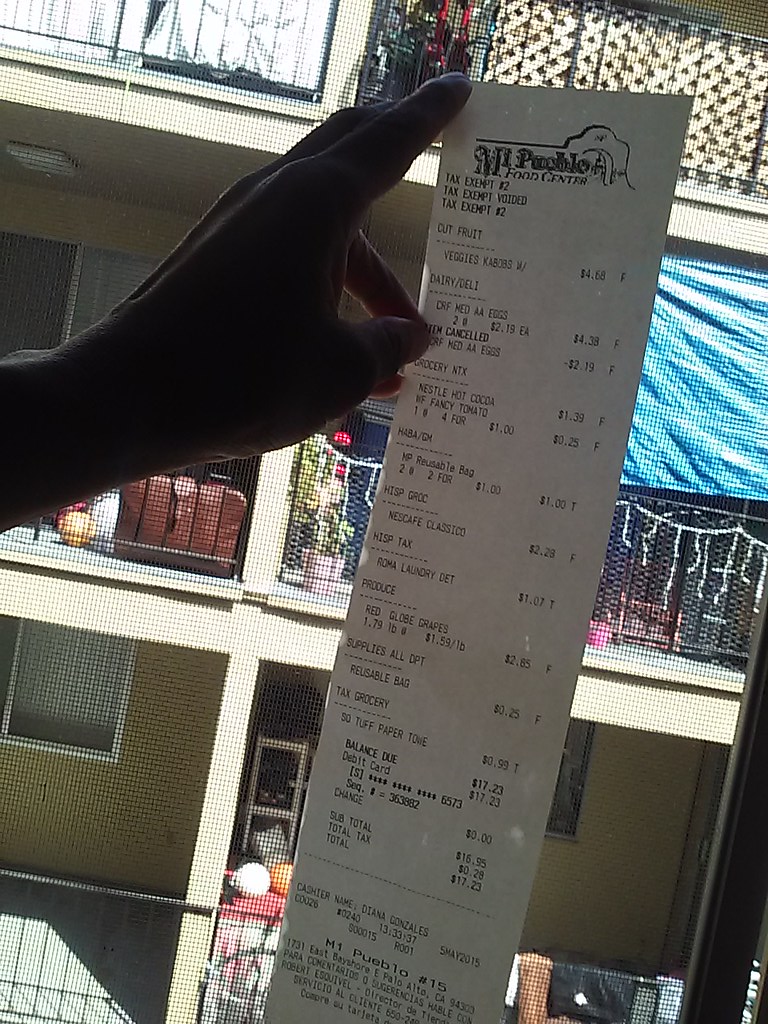A detailed photo caption of a lengthy grocery store receipt held up against a window screen. The receipt, from MT Pueblo Food Center, lists various items including cut fruit, veggie kebab, dairy/deli, and Nescafe Classico, along with a note indicating the shopper is tax-exempt. The cashier's name, Diana, and store number, 15, are also visible. In the background, the window screen reveals glimpses of neighboring apartment buildings and balconies, with one porch adorned with Christmas lights, adding a festive touch to the scene.